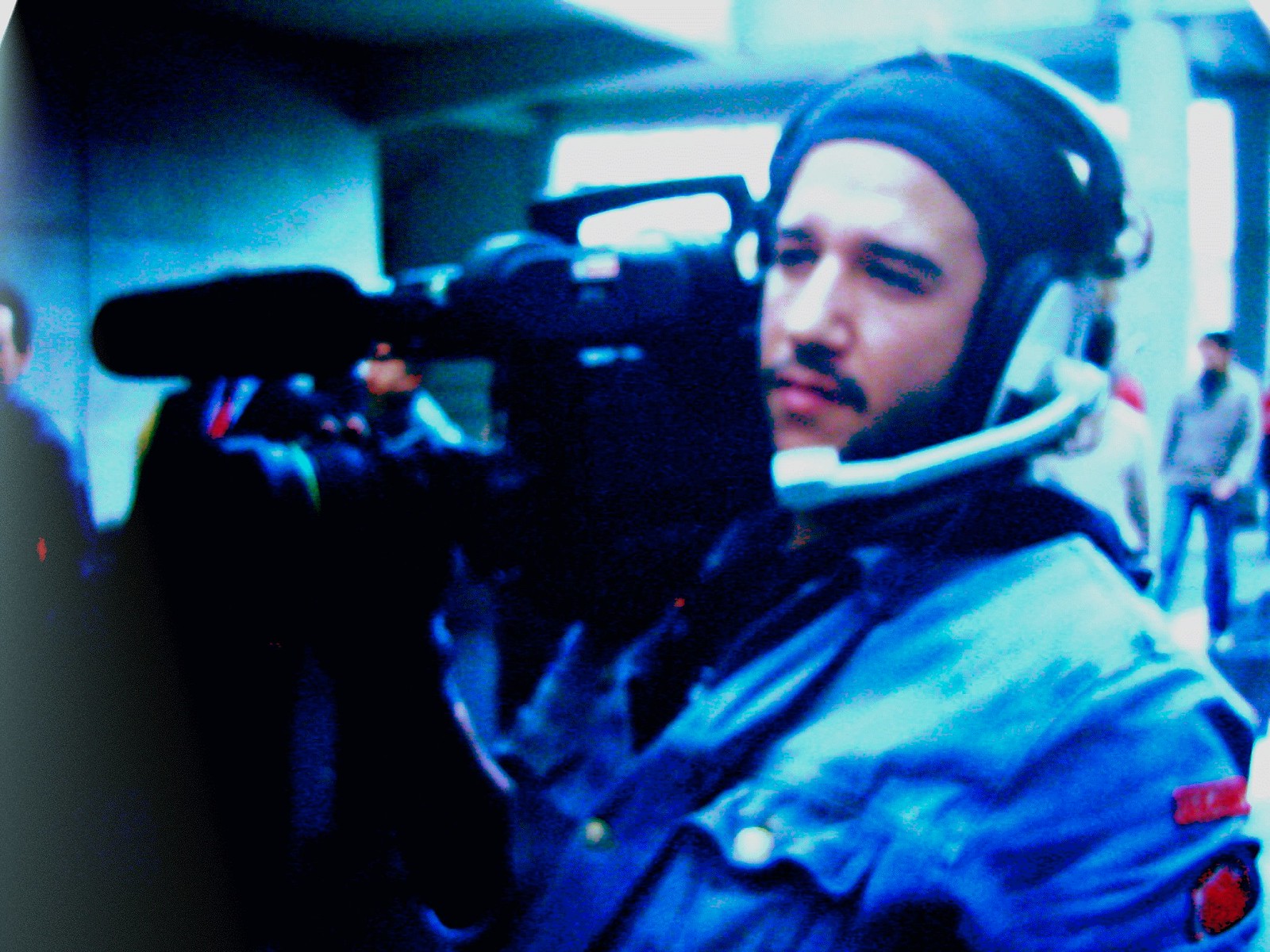This image captures a very blurry and dark scene featuring a bearded and mustachioed cameraman as the primary subject. The cameraman, who appears off to the left, is shouldering a large, expensive camera with a prominent microphone attachment. He is dressed in a blue jacket with a red patch on his left elbow, a beanie, and a chunky white headset equipped with earmuffs and a microphone that extends in front of his mouth. The background, although indistinct, suggests an outdoor, possibly urban, setting with hints of people walking and a building pillar visible in the top right corner. The overall graininess and low light of the photo make it difficult to discern finer details.